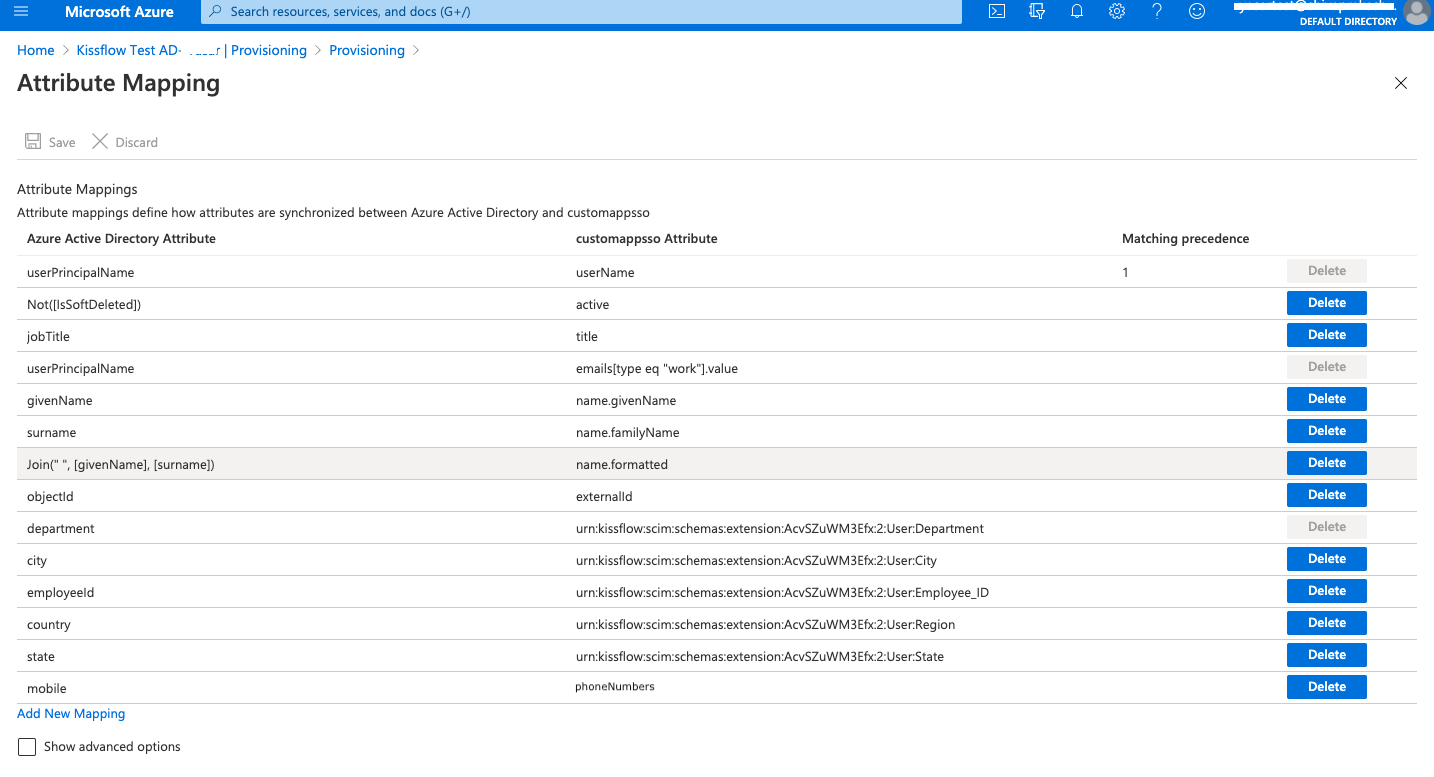This image displays an attribute mapping page in the Microsoft Azure portal. The top of the page features a blue header bar with "Microsoft Azure" prominently written across it. To the right, a search field is labeled "Search resources, services, and docs...", accompanied by five or six icons; however, the specific icons are indistinguishable except for one that appears to resemble a settings menu.

Below the header, the main content is titled "Attribute Mapping." The navigation path displayed includes "Home," "KISSflow Test," "AD," "Provisionings," and "Provisioning." Underneath, a sub-header reiterates "Attribute Mapping" alongside two action buttons labeled "Save" and "Discard."

A brief instructional text indicates that "Attribute Mappings define how attributes are synchronized between Azure Active Directory and another system," although the latter part of the sentence is partially obscured.

The content is organized into three primary columns: "Azure Active Directory Attribute," "Custom App Attribute," and "Matching Precedence." Due to small text size, the specific details within these columns are not readable, though they seem to include elements like File Paths and potentially other types of attributes. The rightmost column contains several delete buttons, most of which are blue with a few in white, aligned with various rows.

Overall, each row is separated by horizontal gray lines, providing visual distinction, although some rows are highlighted with different colors for unspecified reasons.